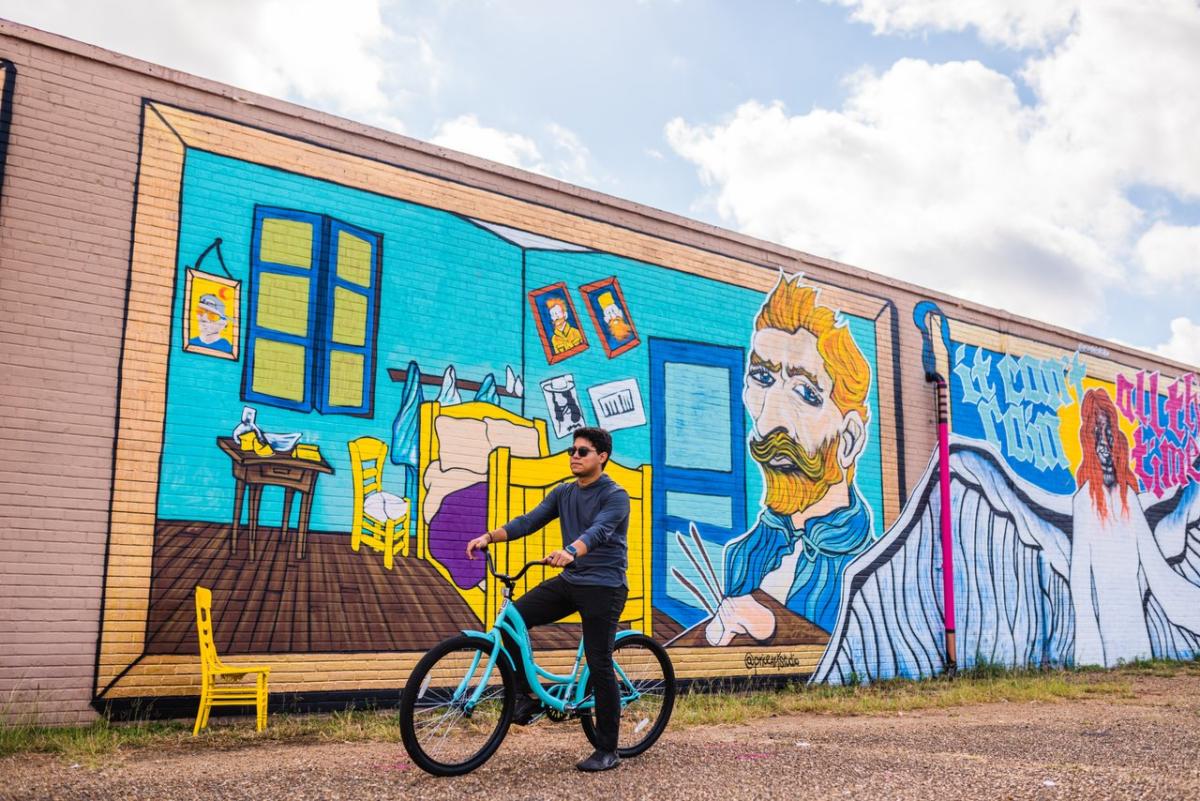In this vibrant outdoor photograph, a young man poses on a blue bicycle with one leg down, in front of a striking mural that blankets the tan brick surface of a large commercial building. The mural, rendered in bright hues, predominantly showcases a detailed depiction of a bedroom scene. The walls of the room are painted turquoise blue, accented by a wooden planked floor, a yellow bed with a purple blanket, and several crooked hanging artworks. Dominating the right side of the mural is a tremendously large bust of a man resembling Van Gogh, with orange hair, a beard, and a blue coat, gazing contemplatively to the side. Near the bed, a small yellow wooden chair and a shaker-style table add depth to the artwork. Additional furniture, including a matching chair positioned on the ground in front of the mural, complements the scene. To the right of this bedroom vignette, another mural features a white angelic figure with demonic red hair and a partially illegible text that seemingly reads "it can't all the time." The vivid blue sky and scattered white clouds lend a serene backdrop to this creative urban tapestry.